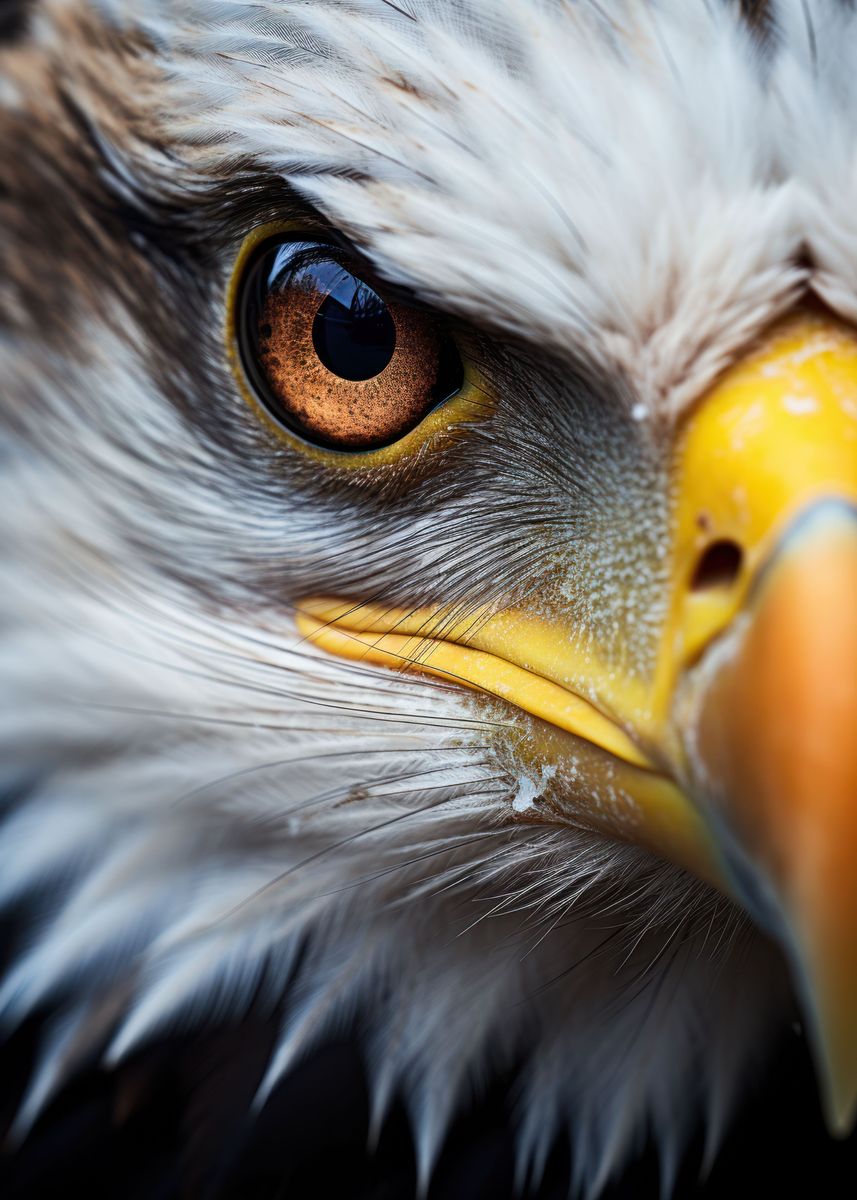This is an incredibly detailed, close-up photograph of the left side of a bald eagle's face, possibly enhanced or AI-generated given its almost unrealistic definition. The focus is on the eagle's intense, copper-colored eye, framed by a narrow yellow ring and underscored by a sharp, scowling brow. The eagle's hooked beak is prominent on the right side of the image, with its yellow base transitioning to an orange-tipped point. The close-up depth reveals white feathers on the head, with some brown feathers visible near the back of the eye and down on the chest. Notably, there is no visible background, emphasizing the high-resolution details of the eagle’s face and giving it a determined, almost menacing expression.